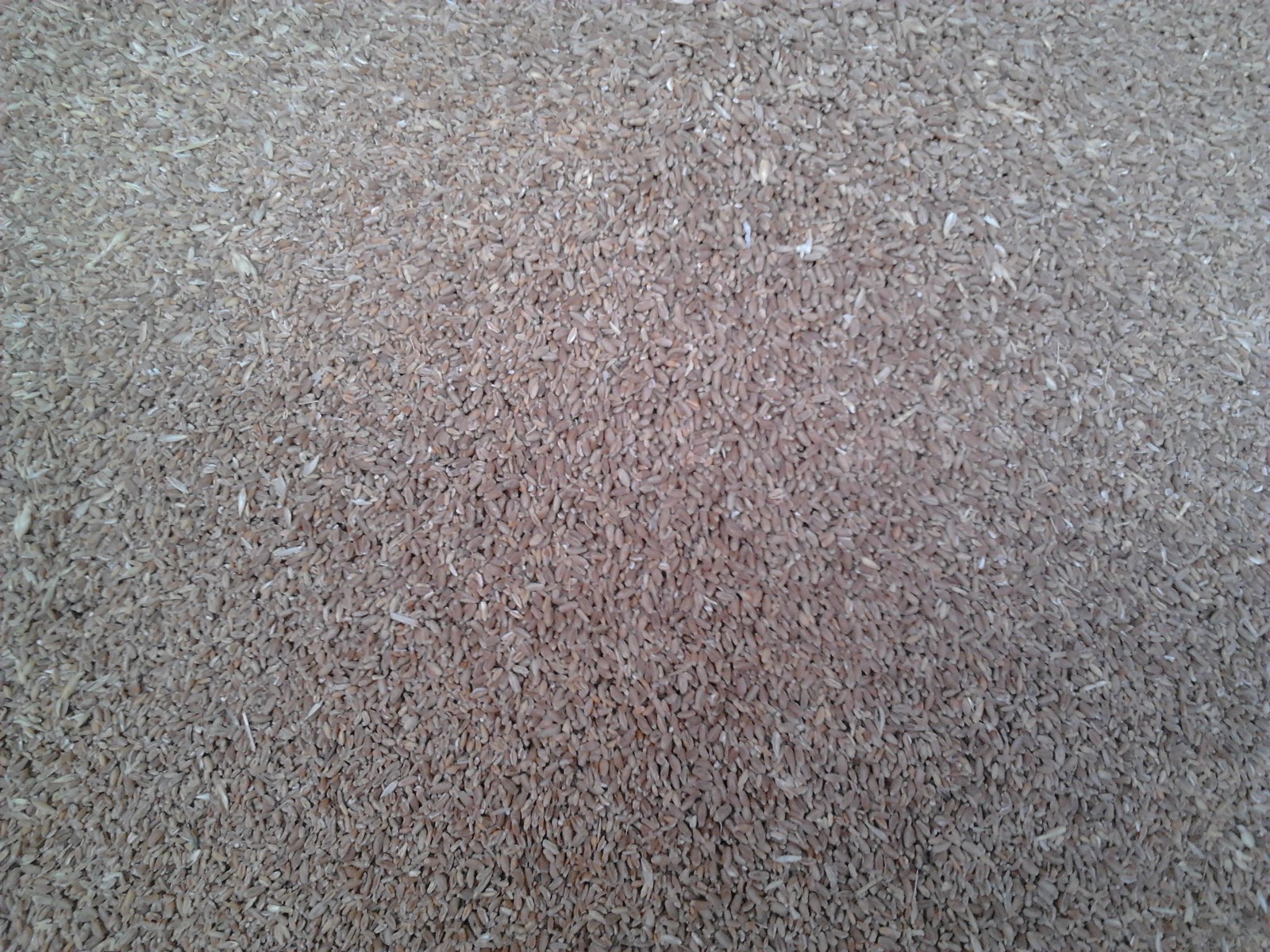This image depicts a tightly focused, zoomed-in shot of an indistinguishable pile, possibly of mealworms or grains of rice, characterized by a mixed texture that could also resemble shredded paper or sand. The entire frame is filled with countless small, tan, light brown, and white particles, with no other objects or text present in the image. It is unclear whether the photo was taken indoors or outdoors, and due to the close-up nature of the shot, the setting is indeterminate. The material forms a continuous, dense pile, and the photograph is either taken from directly above or at a slight angle, focusing exclusively on the granular texture and color of the objects.